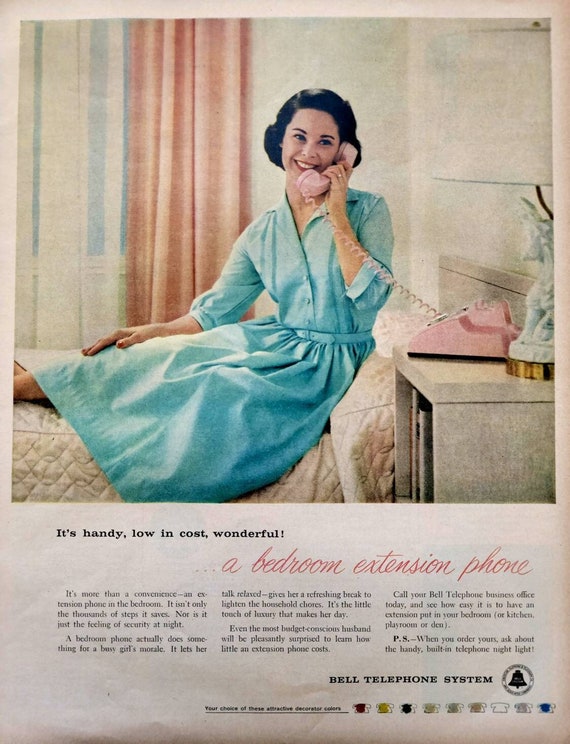This is a vintage magazine clipping, most likely an advertisement from the Bell Telephone System dating back to the 1950s. The page, which has a worn, brownish hue of aged paper, features a large, evocative photograph of a cheerful housewife seated in bed. The woman, dressed in a pleated blue dress with a small belt, sports a classic 1950s hairstyle—short, combed over to one side with a permed look, complemented by red lipstick and red fingernail polish. She is holding the pink receiver of a rotary phone, which rests on a white nightstand beside her. Behind her are peach and white curtains. The setting is cozy and evocative of a mid-century bedroom. The bigger, italicized text beneath the image emphasizes "a bedroom extension phone" with an accompanying slogan in smaller text, reading, "handy, low in cost, wonderful." Columns of text below further extol the virtues of the phone, humorously noting that having a bedroom phone enhances a busy girl’s morale by allowing her to converse in a relaxed manner. The overall aesthetic and detailed advertisement represent a nostalgic glimpse into mid-20th-century domestic life.